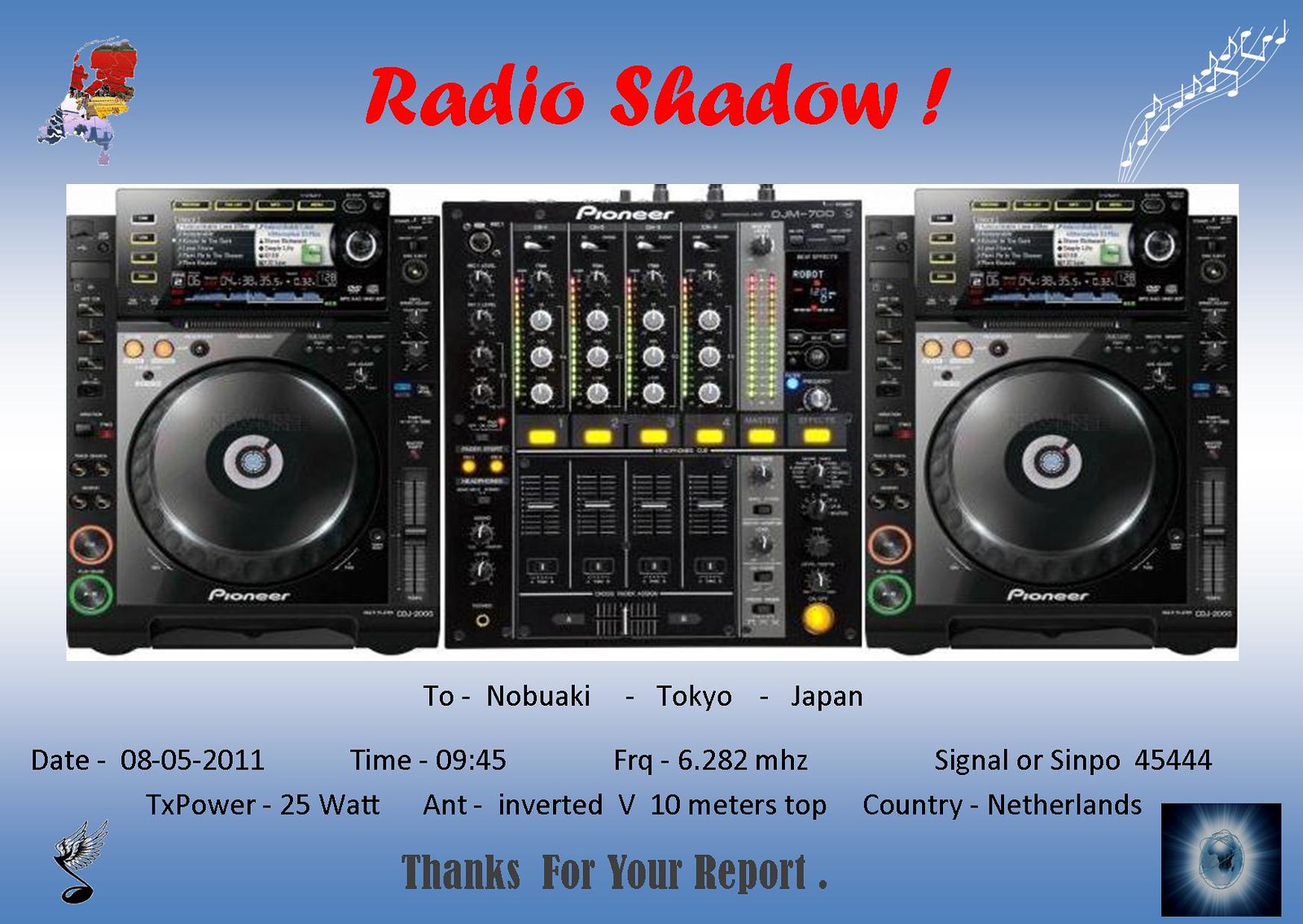This advertisement for a radio show, "Radio Shadow!" features a striking blue and white background. Dominating the top of the image, the show's title is emblazoned in bold red letters, accompanied by an exclamation point. In the top left corner, a multicolored logo, perhaps a stylized profile of a human head, adds a burst of red, yellow, blue, and white hues.

Central to the image is a close-up view of a Pioneer portable stereo with its notable brand name displayed in small white letters. The stereo boasts an array of features including several rows of dials and switches, as well as six yellow indicator lights, all accompanied by two detachable circular speakers positioned on either side. White musical notes, depicted on a curved staff, ascend diagonally in the top right corner, adding to the musical theme.

Beneath the stereo, detailed information is provided in black text: "To Nobukai, Tokyo, Japan." Below this, further specifications are listed, including a date "8/5/2011", time "9:45", frequency "6.282 MHz", signal rating "SENPO: 5444", TX power "25W", antenna type "inverted V, 10 meter", and the country as "Neanderthals". At the bottom of the image, a message of gratitude reads, "Thanks for your report."

Additional distinctive elements include a music note with wings in the bottom left corner and a luminescent egg in the bottom right, adding a whimsical touch to the image.